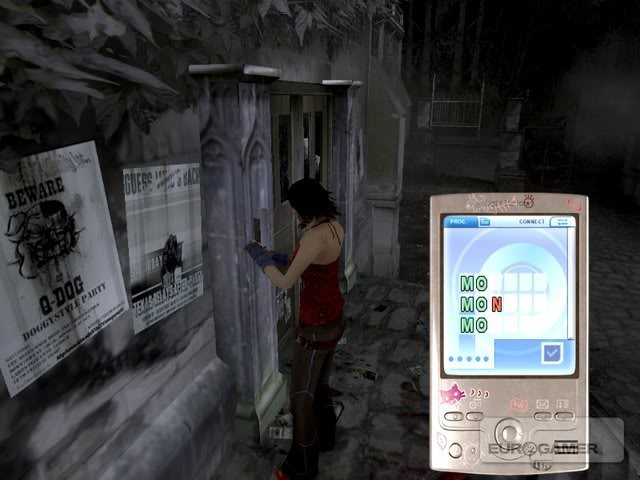This screenshot is from a highly detailed video game, capturing an industrial street scene at night. The atmosphere is dark and immersive, featuring realistic textures and lighting that enhances the night-time setting. In the bottom right corner, a silver device resembling a phone or remote control is prominently displayed, with the text "Mo Man Mo" visible on its screen. Overlaid on this device is the translucent logo of "Eurogamer."

Central to the scene is a lone figure, positioned with their back to the viewer. The figure's appearance is distinctive, with dark black hair, blue gloves, a red shirt, and a contemplative stance that suggests they are engaged in a covert or significant activity. The setting is further enriched by two notable posters affixed to the building wall in the background; one reads "Beware G-Dog," while the other simply says "Guess," though neither are fully legible beyond these words.

The visual style of the scene is reminiscent of modern open-world games such as the Grand Theft Auto series, characterized by its detailed urban environment and realistic portrayal of night-time activity.